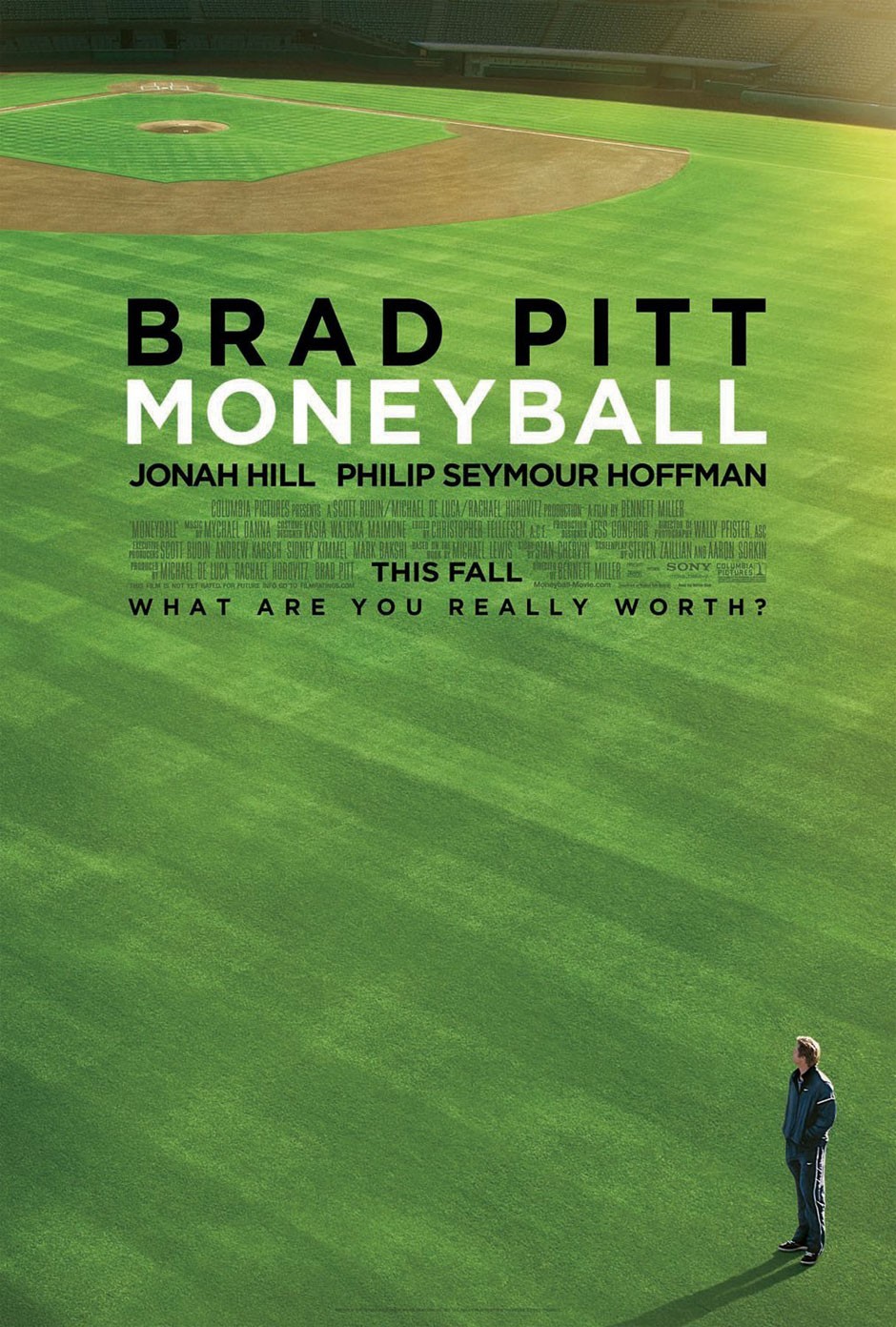This intricate poster for the movie "Moneyball" prominently features an expansive, empty baseball field characterized by its meticulously mowed crisscross patterns, exuding a vibrant spring green. The scene is set against the hint of an empty stadium, complete with bleachers, dugouts, and seats receding into the background. In the bottom right corner of the poster, a solitary figure, identified as Brad Pitt, stands in a track suit, looking towards home plate, emphasizing the vastness and solitude of the field.

The textual elements are clean and distinctly laid out in a blocky, sans-serif font. At the top center, "Brad Pitt" is boldly displayed in black, followed by the movie title "Moneyball" in prominent white. Beneath the title, the names Jonah Hill and Philip Seymour Hoffman appear in smaller black text, with additional cast and production credits detailed further down. The poignant tagline "What are you really worth?" invites introspection, nestled at the bottom of this evocatively simple yet engaging poster.